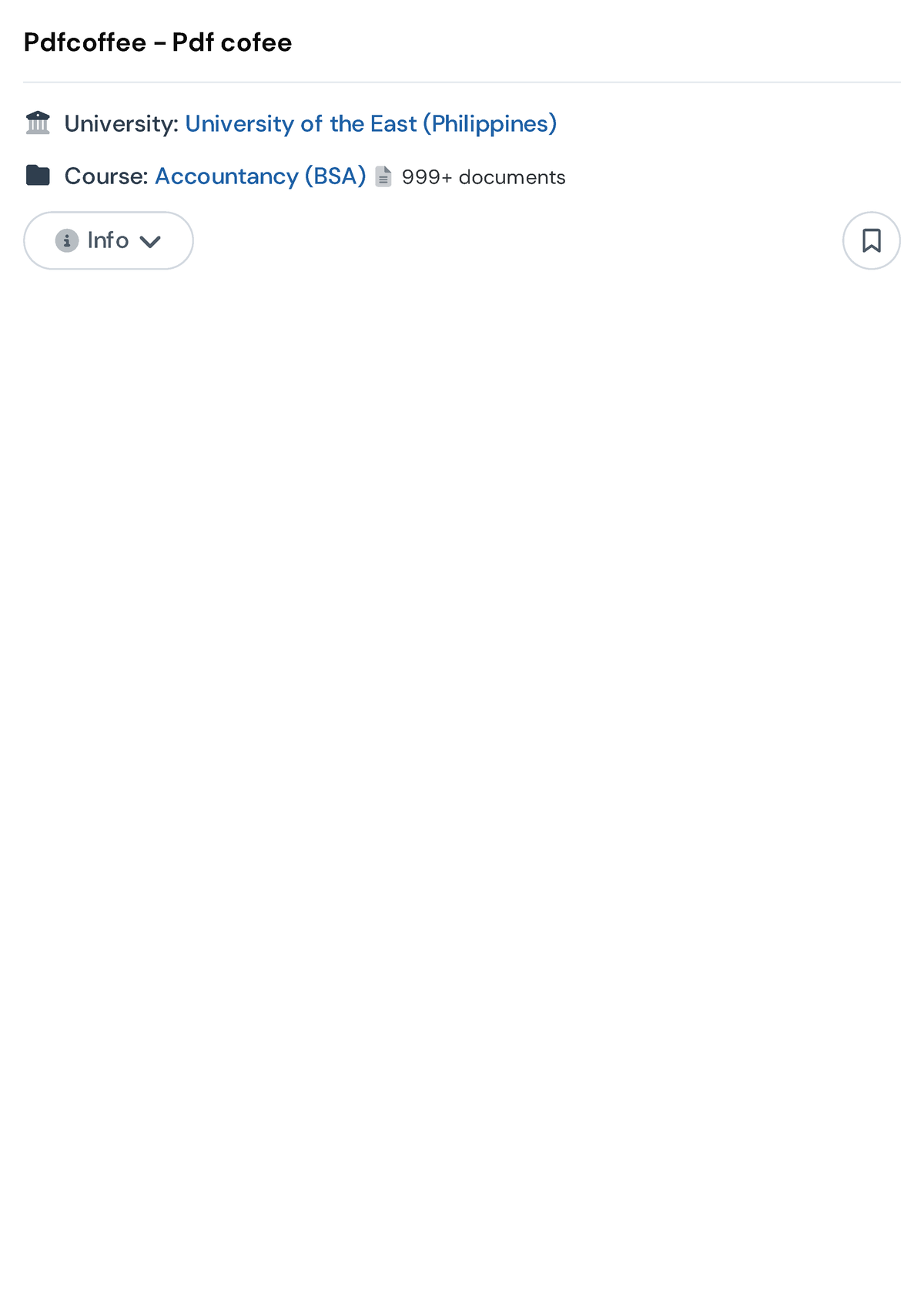This image is a compact screenshot featuring the header of a PDF file of a resume. The header begins with "pdfcoffee - pdf coffee" where "pdfcoffee" is written all in lowercase with two 'f's, and "pdf coffee" has only one 'f'. Below this header text, there's a thin gray separator line. Underneath the line, there is a small icon labeled "university." To the right of this icon, the text "University of the East Philippines" is written in blue, suggesting a clickable hyperlink.

Below the university information, another icon resembling a folder appears. To the right of this folder icon, the word "course" is displayed. Next to "course," the specific field of study "Accountancy (VSA)" is mentioned. Further to the right, the text "999+ documents" appears in small gray letters, indicating a substantial number of documents associated with the course.

Below this section, there is a round button labeled "info" with a downward-pointing arrow to its right inside the button. On the far right side of the header, a small white circle containing a bookmark icon is visible. The remainder of the page shown in the screenshot is blank.